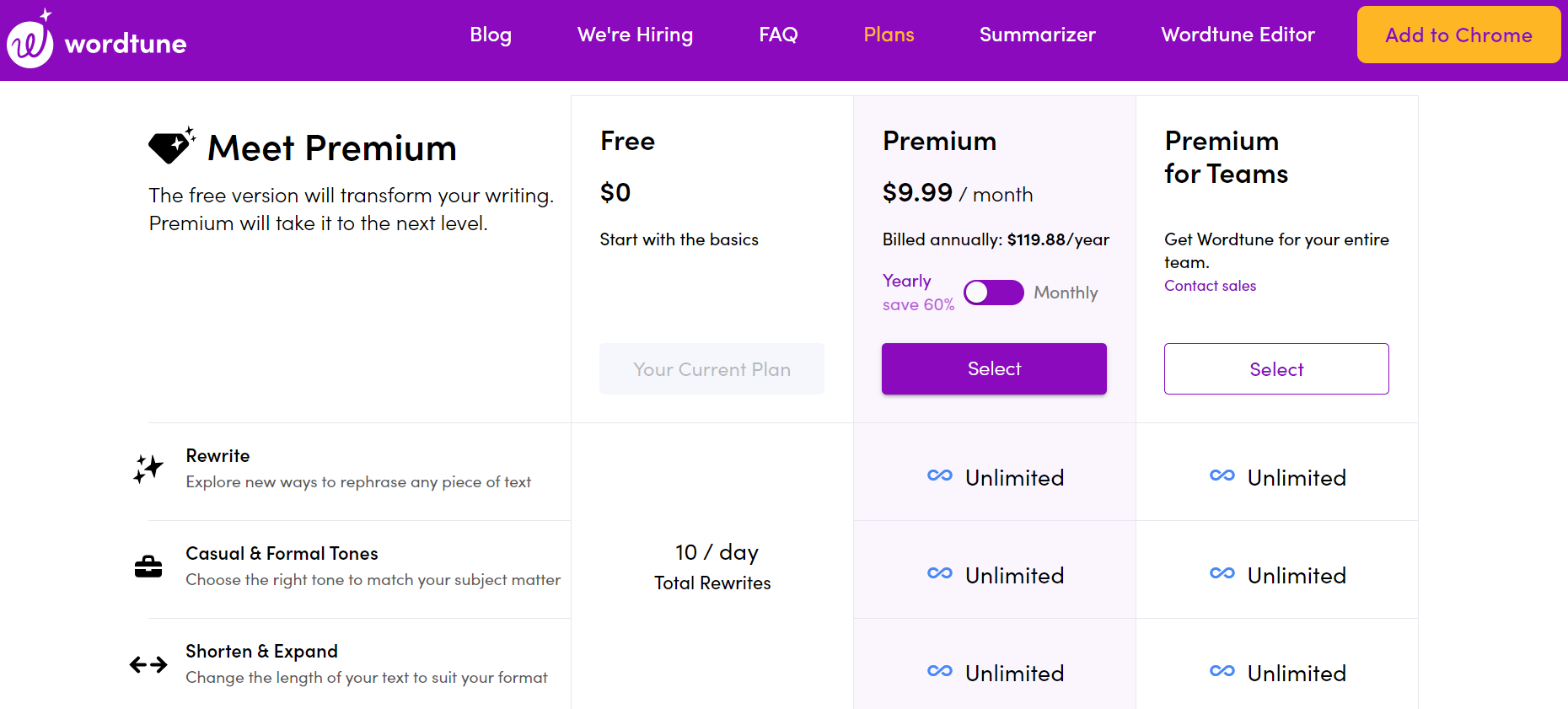The website showcases different purchasing plans for the WordTune software. The logo features a white circle with a purple, handwritten "W" on a dark purple header that transitions from left to right. In this header, options including "Blog," "Careers," and "FAQs" appear in white text. One of the purchasing plans is highlighted in yellow, and there is a button on the far right side that says "Add to Chrome," written in purple on a yellow tab.

Below the header, on the far left, an announcement marked with a diamond symbol introduces the Premium plan. The announcement reads, "Meet Premium: The free version will transform your writing, premium will take it to the next level."

The plans are detailed as follows:

- **Free Plan**: Costs $0 and is listed as the current plan for the individual. It includes basic features with a limitation of 10 total rewrites per day.
  
- **Premium Plan**: Costs $9.99 per month if billed annually, totaling $119.88 per year with a 60% savings when you choose the yearly billing option. This plan includes unlimited access to all features such as rewriting, casual and formal tones, shortening, and expanding text.

- **Premium for Teams**: Designed for organizations, this plan does not list a specific cost. Instead, it encourages users to contact sales for pricing details. This option also offers all features with unlimited access.

These detailed purchasing plans are aimed to cater to individual users and teams, providing various levels of functionality to enhance their writing experiences.